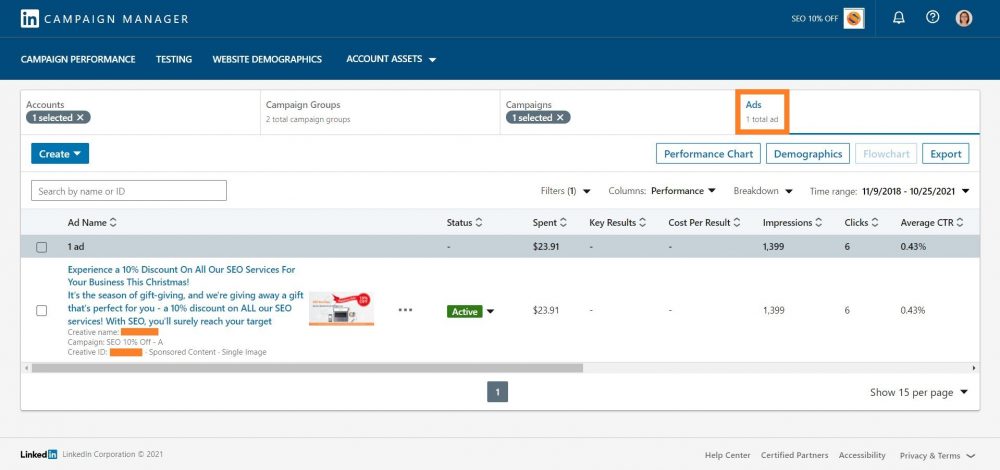The image is a screenshot of an application interface specifically designed for a campaign manager on LinkedIn. In the top left corner, there is a recognizable LinkedIn logo inside a white square, labeled "IN," and next to it, the text "Campaign Manager" is prominently displayed. The interface is divided into several sections including "Campaign Performance," "Testing," "Website Demographics," and "Account Assets."

In the top right corner, there is a promotional banner reading "SEO 10% off," followed by a notification icon, a help icon indicated by a question mark, and a user profile icon displaying a picture of the person’s face. Below this bar, the text "Account Selected: One account selected" is shown, and it indicates that no specific campaign is currently selected.

Further down, the interface lists "Campaign Groups," noting "Two Total Campaign Groups," with one campaign being selected. 

A highlighted banner below the campaign group section advertises, "Experience a 10% discount on all our SEO services for your business this Christmas. It's the season of gift-giving and we're giving away a gift that's perfect for you, a 10% discount on all SEO services. With SEO, you'll surely reach your target."

Following this, there is a section labeled "Creative Name," with its content concealed by an orange box, and "Campaign: SEO 10% off" is displayed underneath. The "Creative ID" is also obscured by an orange box. Next to these details, there is a small, indiscernible image related to the campaign product. 

At the bottom of the section, there is a drop-down menu marked "Active" in a green box, and a financial detail showing "$23.91."